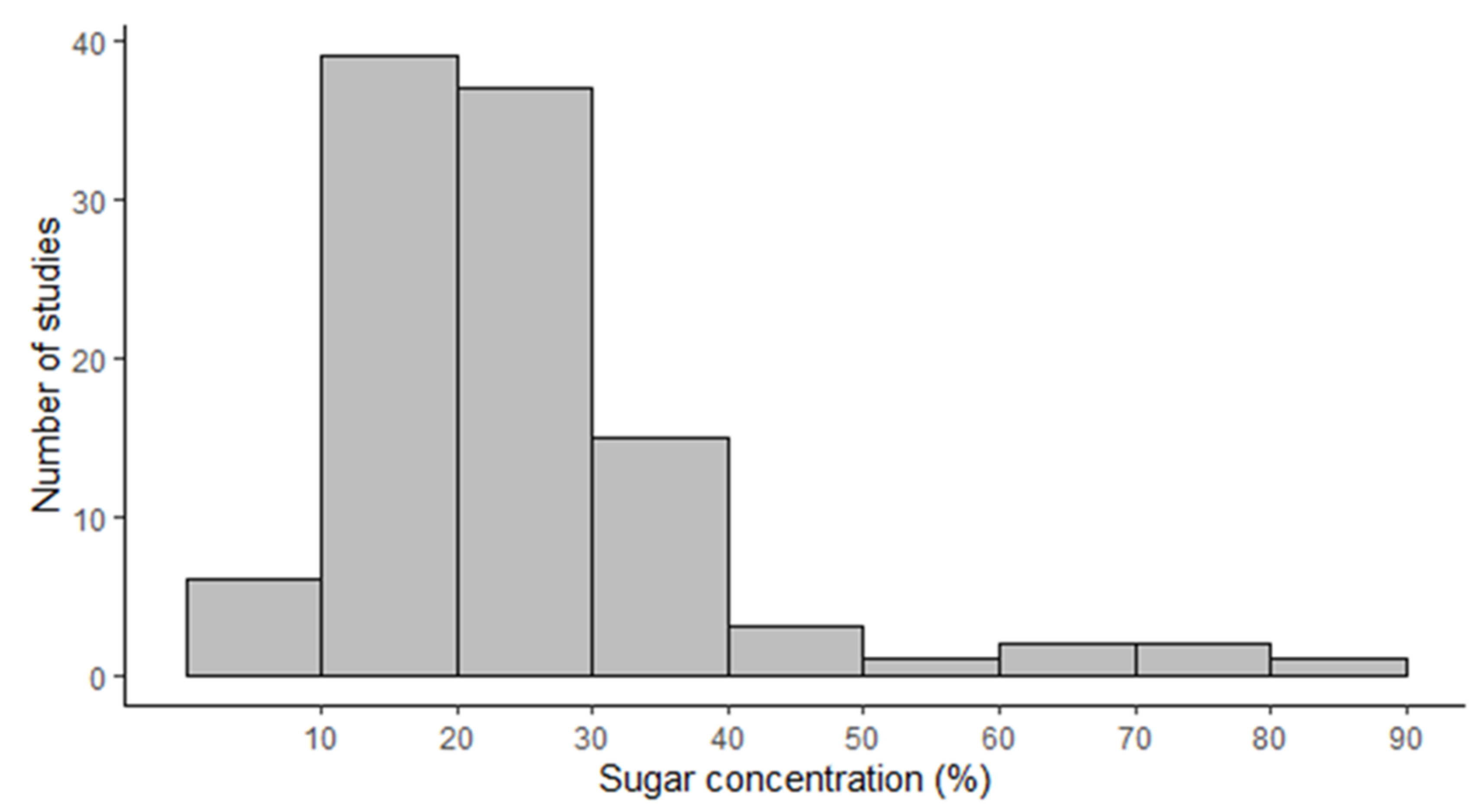The image depicts a bar graph on a white background, with black outlines and labeling. The y-axis is labeled "Number of Studies" and is marked in increments of 10, ranging from 0 to 40. The x-axis is labeled "Sugar Concentration (%)" and is marked in increments of 10, ranging from 0 to 90. Each bar in the graph is filled in gray. The bars illustrate the number of studies corresponding to different sugar concentration percentages as follows:

- The first bar, representing 0-10% sugar concentration, reaches approximately 5 studies.
- The second bar, for 10-20% sugar concentration, peaks at around 38 studies.
- The third bar, covering 20-30% sugar concentration, slightly declines to about 37 studies.
- The fourth bar, indicating 30-40% sugar concentration, drops significantly to approximately 12-15 studies.
- The fifth bar, for 40-50% sugar concentration, shows roughly 4 studies.
- The sixth bar, representing 50-60% sugar concentration, illustrates around 2 studies.
- The seventh and eighth bars, covering 60-70% and 70-80% sugar concentrations respectively, each show about 3 studies.
- The final bar, representing 80-90% sugar concentration, shows approximately 2 studies.

This detailed representation highlights the variations in the number of studies conducted across different sugar concentration levels.